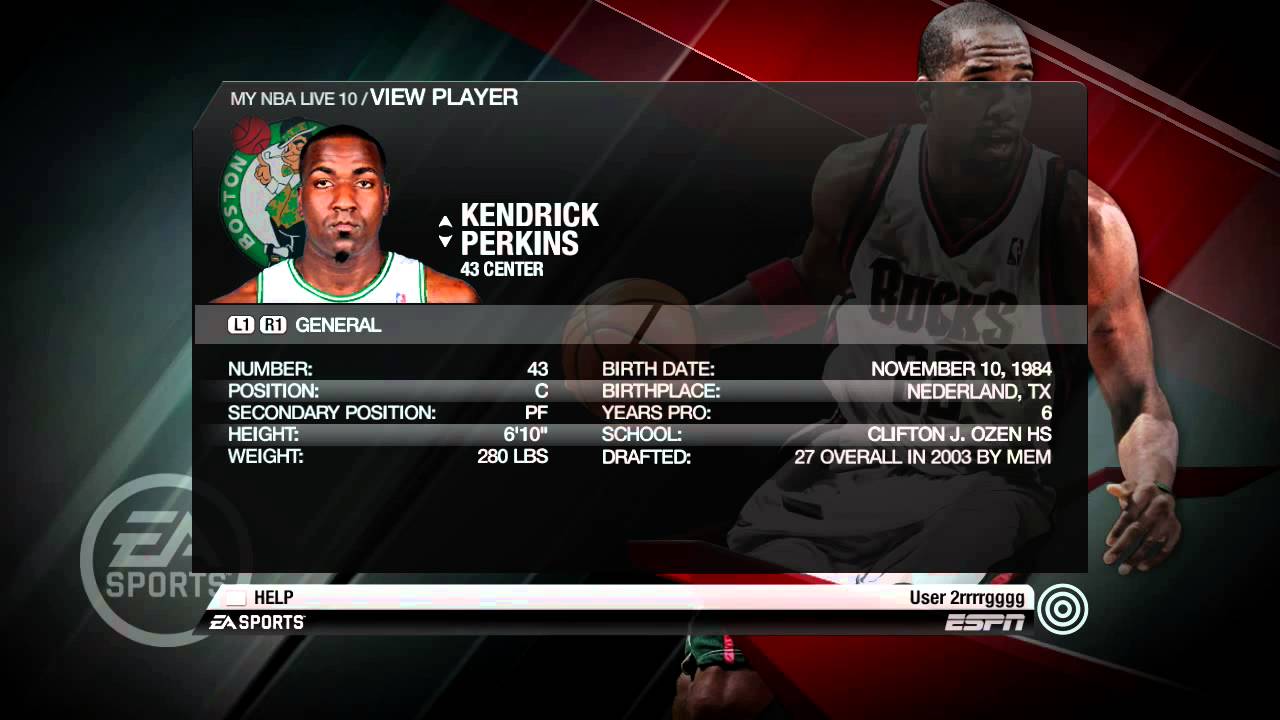This detailed caption describes an NBA Live action figure of Kendrick Perkins, the center wearing jersey number 43. Standing at 6'10" and weighing 280 pounds, Perkins was born on November 10th, 1984, in Nederland, Texas. He spent 6 years as a pro after being drafted 27th overall by the Memphis Grizzlies in 2003, hailing from Clifton J. Ozen High School. The detailed figure includes secondary position credentials as power forward (P.F.), labeled as "L1R1 General." The box art features a whimsical leprechaun spinning a basketball on his finger, promoting Boston's team spirit. Perkins is showcased in his white and green Boston Celtics jersey, highlighted by EA Sports and ESPN branding.